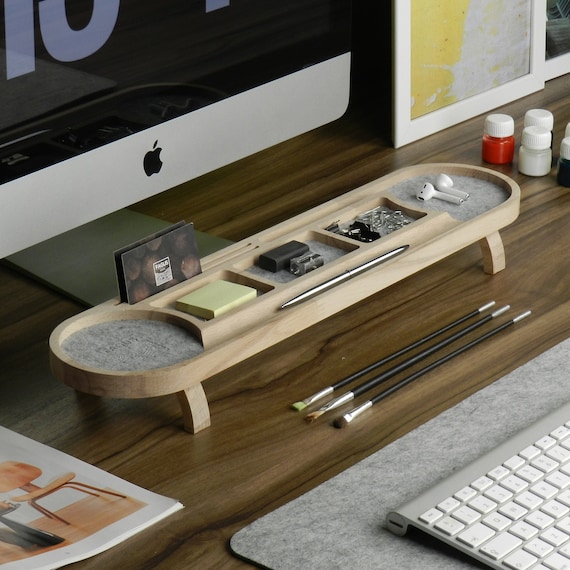This image depicts a meticulously organized workspace. At the heart of the scene is a medium-toned brown wooden desk. Dominating the upper left corner is the lower half of an Apple monitor, identifiable by its silver base and signature logo. The screen is barely visible but seems to display a black interface with white graphics. 

In front of the monitor sits a racetrack-shaped wooden organizer tray. This light wood tray features compartments, holding various desk tools: paperclips, yellow sticky notes, a pen, what appears to be an eraser and a pencil sharpener, and a pair of Apple AirPods. The tray ends are accentuated by gray felt pads.

Directly in front of the tray, three paintbrushes with black handles and gray tips are aligned neatly on the desk. To the right of the tray, small circular glass bottles filled with paints—red, white, and black—are arranged with white caps reflecting the light.

Further to the right, a sleek Apple keyboard with white keys rests on a matching gray felt mat. This mat mirrors the soft tones of the felt pads on the organizer tray, tying the desk elements together in a cohesive aesthetic.

In the upper right, additional art supplies, including more small paint bottles, add to the creative ambiance of the workspace. The lower left corner slightly reveals a framed photo or a painting showcasing hues of yellow and white, adding a personal touch to the scene.

Overall, this detailed snapshot of a creative individual's desk highlights their orderly arrangement of both digital and traditional art tools, blending technology and artistry harmoniously.